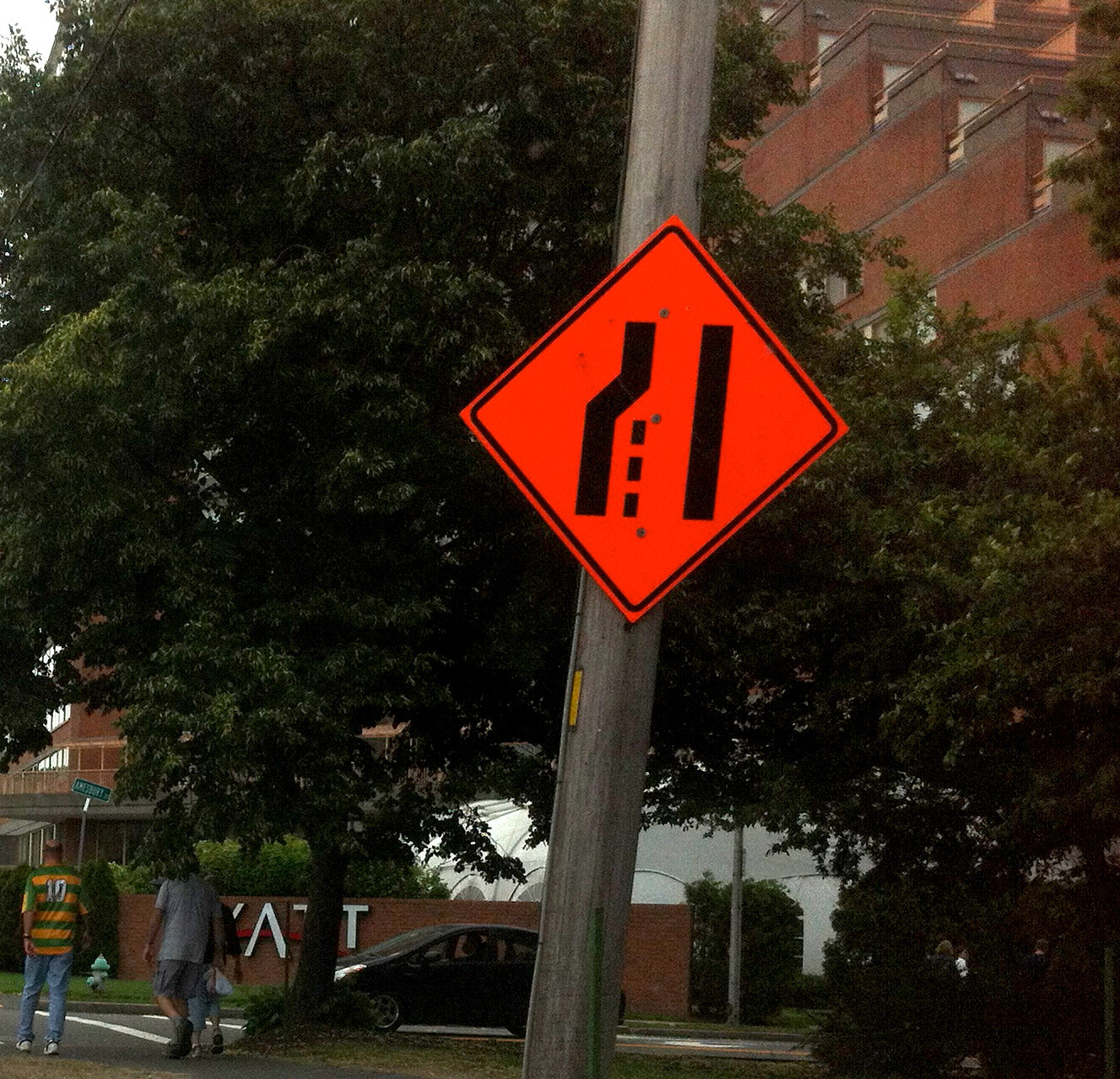The image depicts an orange, diamond-shaped merge sign with black lines indicating a lane narrowing on the left side, mounted on a wooden pole. In the background, mature, leafy trees provide shade in front of a red brick building that ascends in a step-like fashion, possibly a hotel or an apartment block. The building's red brick wall features partial white lettering, potentially spelling out "Hyatt." At the bottom left, three people are visible: one in a green and yellow t-shirt with white number '10' on the back, blue jeans, and white sneakers; another in a grey t-shirt with dark grey shorts; and a third in a darker top with light blue jeans. They appear to be crossing the road near a black hatchback car. On the opposite side of the road, a blue fire hydrant stands on the grassy sidewalk, adding to the scene's urban detail.